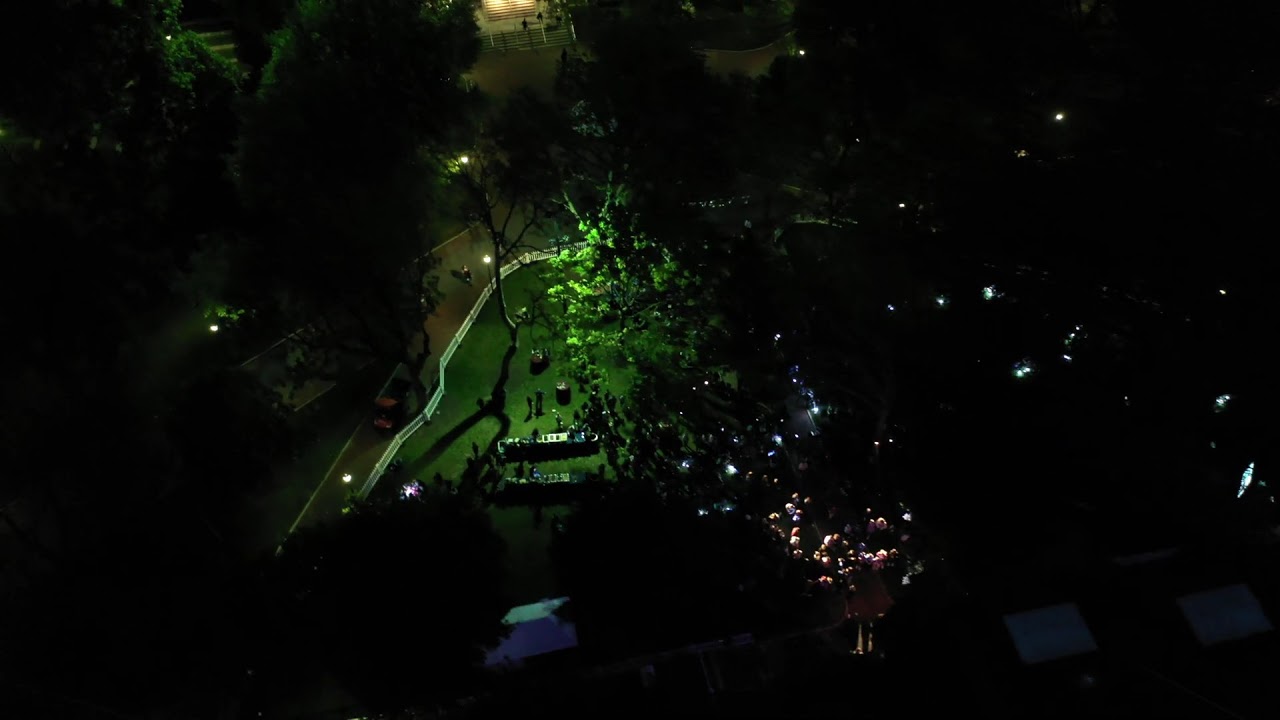This nighttime aerial photograph, taken in color and in landscape orientation, captures a dimly-lit outdoor scene. The majority of the image is cloaked in darkness, with scattered lights illuminating certain areas. Slightly off-center, a white wooden picket fence encloses a grassy area, suggesting a backyard or park, possibly hosting a small gathering or outdoor event. Within this enclosed space, artificial green light creates patches of visible terrain.

At the top center of the image, a flight of stairs descends into the brightly lit open space. Trees border the area, their leaves either fully present or absent, casting shadows and obscuring parts of the scene. A walking path lies just outside the fence, where a person and a vehicle are visible. 

Toward the bottom center, a cluster of small lights, possibly from cell phones or lamps, hints at activity or people congregating. Additionally, several indistinct small structures and a main building appear towards the front of the property, enhancing the complexity of the photograph. The style of the image leans towards photographic representationalism and realism, presenting a detailed and true-to-life drone view of the scene.